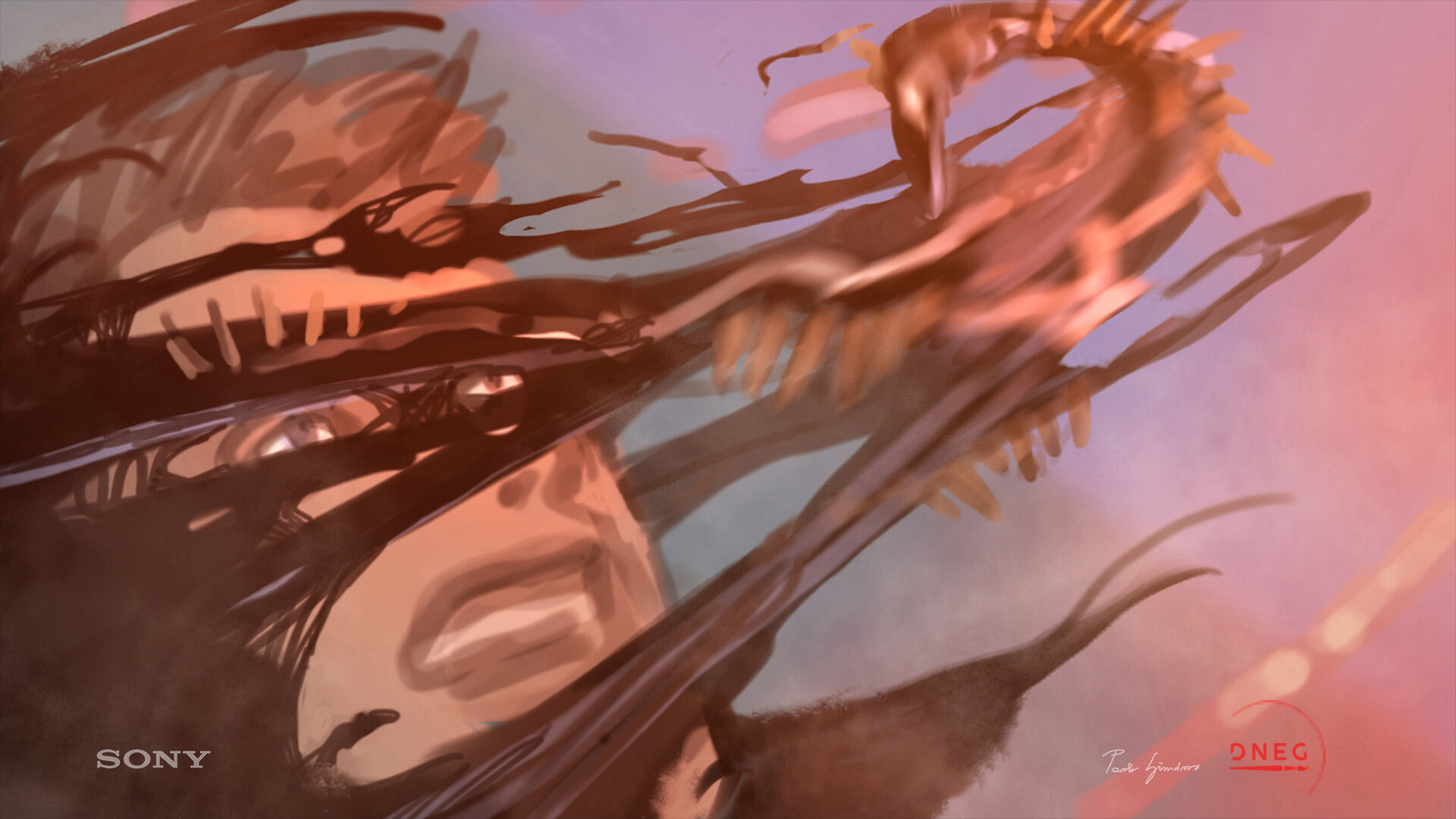The image depicts an intense, digitally animated scene featuring a Caucasian man in his twenties or thirties with blonde, spiky hair and piercing blue eyes. His face conveys a sense of struggle or anger as he grits his teeth, while ominous black tendrils envelop his face, extending over his eyes, nose, and chin. The tendrils, appearing as though they consist of a tar-like substance, stretch outward, merging into the form of a menacing creature that resembles a snake or dragon with glowing eyes, suggesting the presence of the Venom symbiote. The background is a mix of fuzzy, faded colors—reddish, bluish, and greenish—giving an ethereal, cloudy feel. The orientation of the image is horizontal, with “Sony” written in white font in the bottom left corner and “D-N-E-G” alongside an unintelligible cursive signature in red font on the bottom right, indicating its connection to the Venom cinematic universe.